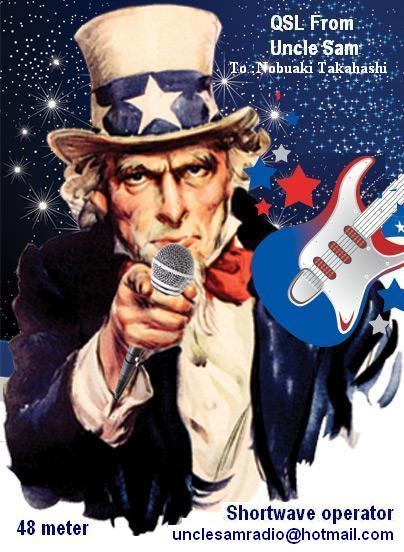The image is a digitally modified poster of Uncle Sam, depicting him in his signature dark blue jacket, white shirt, and red bowtie, with a white top hat that features a blue stripe adorned with white stars. Uncle Sam is pointing directly at the viewer with an intense expression, with a microphone seamlessly integrated into his right hand. On his left shoulder, a red, white, and blue guitar is superimposed, suggesting a patriotic theme. The background is filled with red, white, and blue stars and lights, enhancing the celebratory mood. In the top right corner, text reads "QSL from Uncle Sam to Nobuaki Takahashi." Additional text in the bottom corners includes "48 meter" on the left and "shortwave operator UncleSamRadio at hotmail.com" on the right. The overall styling and elements suggest that the image is promoting a radio channel.